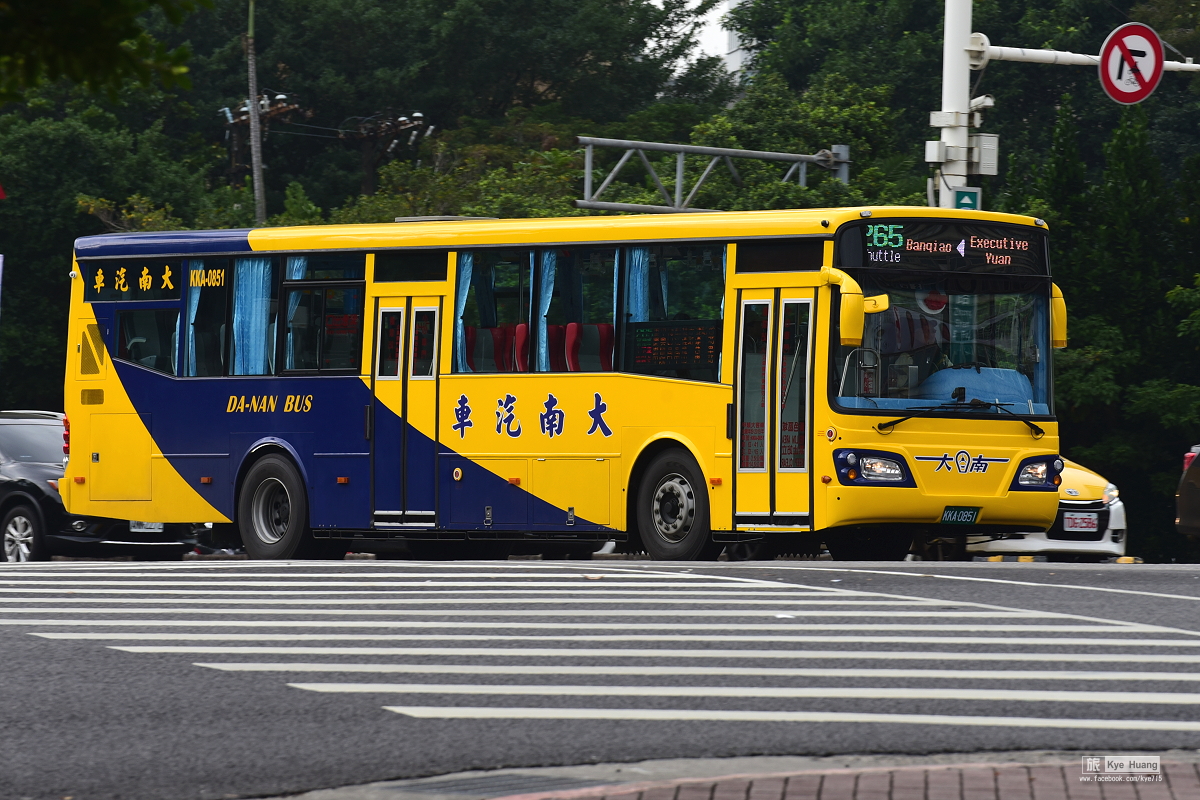This realistic photo captures a bustling city street scene, likely in China. Central to the image is a brightly colored public bus predominantly painted yellow with a distinctive blue streak towards the rear. The blue section of the bus features bold yellow writing that reads "Da Nan Bus," accompanied by Asian characters throughout the exterior. The bus is identified as the 265 Shuttle, with a digital sign displaying "Bangyao Executive Yuan" at the top of its large windshield. The bus has a flat front, two black-framed doors on its right side, and smoked windows with visible high-back red seats and tied-back white curtains. It is stopped at an intersection, evidenced by a prominent white-striped pedestrian crosswalk in the foreground. Surrounding the bus, there is a black car directly behind it and a distinct yellow and white taxi to its right. Additional urban details include street lights, a traffic camera, power lines, and a no right turn sign. The scene is set against the backdrop of a modern city with clear, busy thoroughfares.